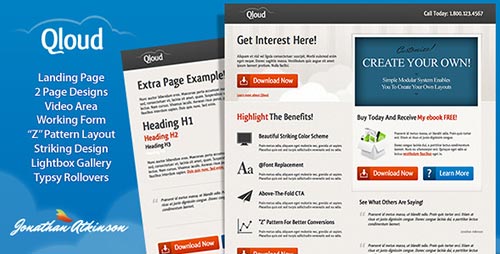This image features the Qloud website, characterized by its blue background and two graphic designs of papers. These papers display various symbols, representing services or products offered by the website. At the bottom left corner, there is a signature by Jonathan Atkinson with a distinctive red logo above it. The background also includes cloud motifs enhancing the visual appeal.

The primary papers are predominantly white with black text, containing advertisements to encourage users to "Get Interest Here" and "Create Your Own." They also prompt visitors to "Download Now" and highlight available benefits. Each paper has a black tab at the top featuring the Qloud logo in white text. Behind the primary paper, an example of an additional page is visible, including an H1 heading underneath it.

The text on the papers has selective use of orange highlights and orange links, along with download buttons to facilitate user interaction. A prominent blue rectangle with a question mark encourages users to learn more. Additionally, the right-side paper showcases an image of a box filled with green items at its center, drawing attention to specific content or offerings on the website.